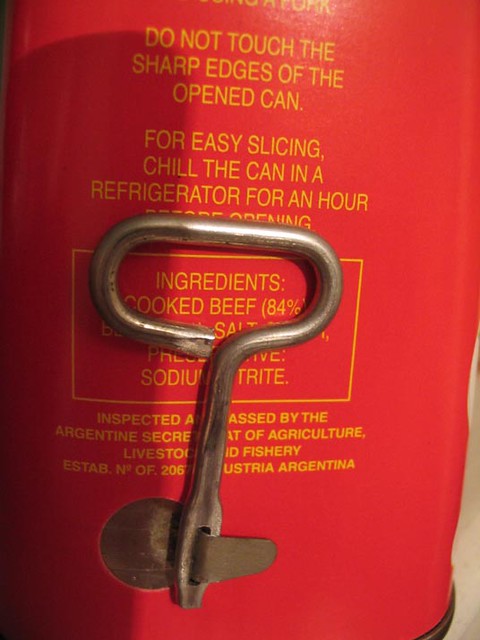A vintage can of Spam is partially visible, showcasing its distinctive red side panel with yellow printing. The label warns, "Do not touch sharp edges of open can. For easy slicing, chill the can in the refrigerator for an hour before opening." The ingredients list reveals that the product contains 84% cooked beef, along with salt and sodium nitrite as a preservative. Some text is obscured, but it's evident that the can has been inspected and passed by the Argentine Secretary of Agriculture, Livestock, and Fishery, with establishment number 0F206, likely in Austria, Argentina or similar. An old-fashioned key mechanism is attached to a metal flap on the can, ready to be turned. This key would peel away a thin strip of metal, allowing the can to be opened and its contents revealed. Such cans were commonly used for potted meats in the past, though they are rarely seen today.